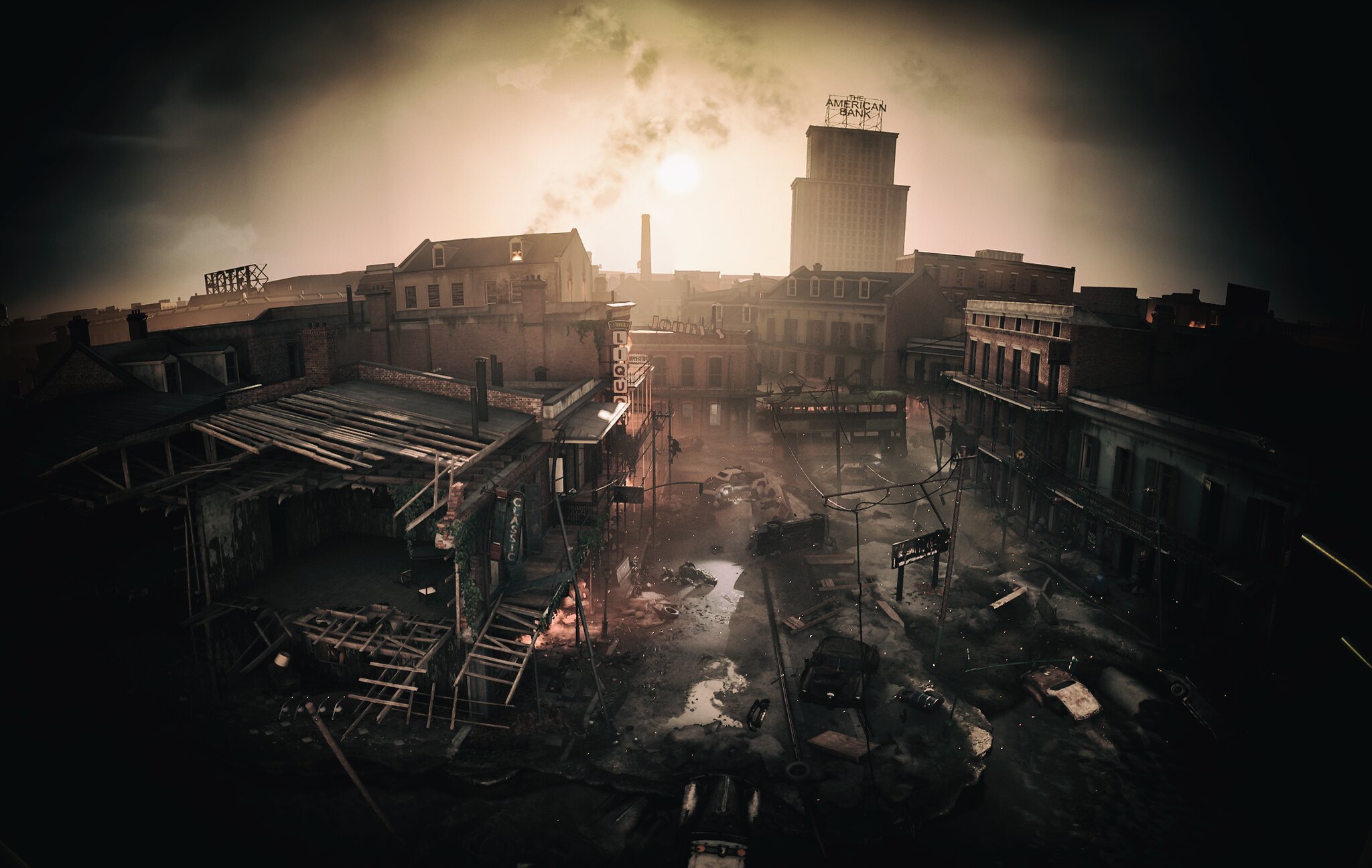This aerial photograph captures a quaint, older town characterized by its historical architecture and laid-back atmosphere. On the left side of the image, there is visible construction activity, with a building undergoing significant repairs. The roof of this building is mostly removed, revealing the exposed board framework. Scattered across the ground, you can observe the framework of walls, suggesting ongoing reconstruction efforts.

Running vertically through the center of the image is a rustic dirt road, adding to the town's nostalgic charm. To the right of this road, a cluster of closely-knit buildings can be seen, showcasing the close community structure typical of older towns. Among these structures is a prominent tall building in the background with the name "American Bank" clearly visible, adding a touch of historical significance to the scene. This blend of old-world charm with the hustle of modern construction portrays a town in the midst of evolution while retaining its heritage.